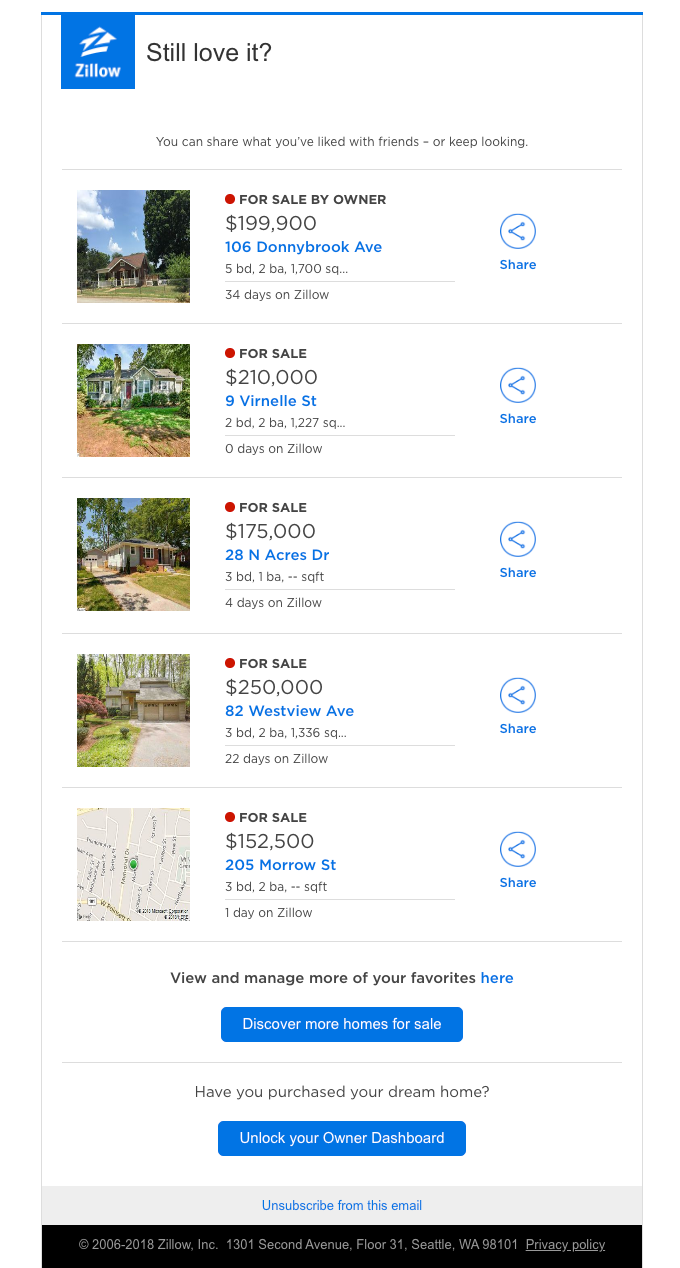This screenshot is from a Zillow webpage. In the upper left-hand corner, a blue square prominently features the white Zillow logo, depicting a small house with a "Z" through the middle. Beneath this logo, the word "Zillow" is inscribed in white text.

Adjacent to the logo, bold black text poses the question: "Still Love It? You can share what you've liked with friends or keep looking." Below this heading, five property listings are displayed in a neat column. The first four listings are accompanied by small photographs of the respective properties, showcasing their exterior or interior. The fifth listing is represented by a small square map with a green pin, indicating the property's location.

For each property, detailed information is provided, including the asking price, address, number of bedrooms, bathrooms, square footage, and the number of days the property has been listed on Zillow. Running down the right-hand side of the page, small share buttons allow users to easily share their favorite properties.

At the bottom of the screen, there is an option to view and manage more of your favorite properties by clicking a link that directs you to a dedicated favorites management page.